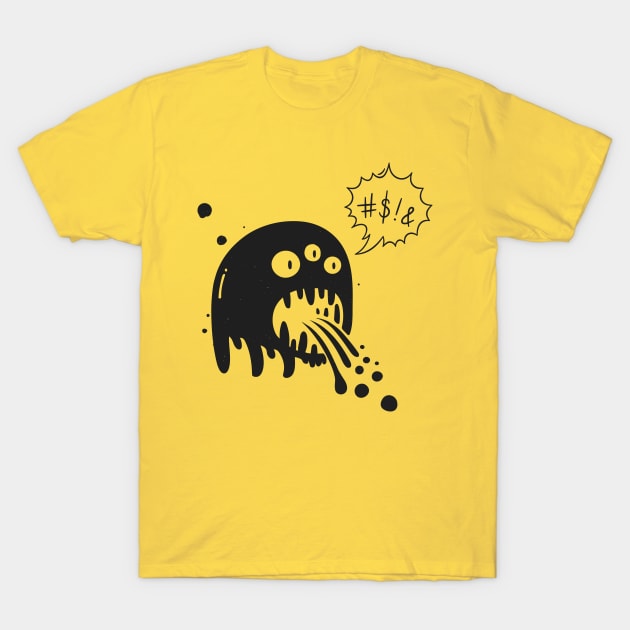This image features a yellow t-shirt laid flat against a stark white background. The shirt, a standard short-sleeved crew neck, is the same hue as a ripe banana. Dominating the front of the t-shirt is a striking black graphic of a cartoony monster. The monster has a blob-like shape, with a dripping bottom edge creating a dynamic look. It has three white eyes arranged asymmetrically: a large one towards the center left, a smaller one slightly above to the right, and another small one further to the right. The monster’s round mouth is open wide, spewing black streaks and dots in a pattern that resembles monster sludge. Adding to the whimsical design, a pointed text bubble filled with symbols (#, $, !, &) hovers above the creature, implying it's swearing. The graphic and its playful, edgy details suggest the shirt is meant to be humorous, ideal for someone seeking a lighthearted, funny fashion statement.